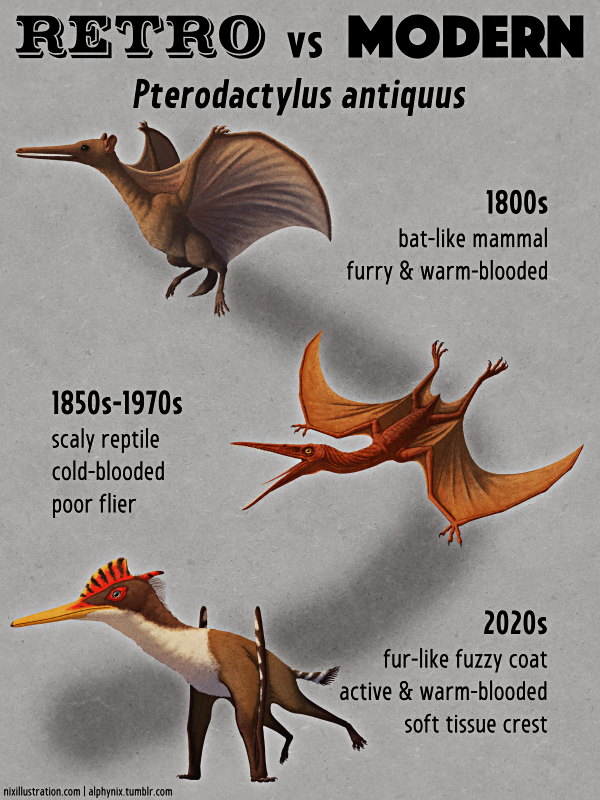The poster, with a chalky gray background, is titled "RETRO vs. MODERN" in bold black, stylized 3D lettering. It features the Pterodactylus antiquus, depicted in three different evolutionary interpretations over time. At the top, the 1800s version of the pterodactyl is shown as a bat-like mammal, furry and warm-blooded. This depiction includes a long-snouted creature with extended wings, raised dog-like ears, and various shades of brown. In the middle section, representing the period from the 1850s to the 1970s, the pterodactyl transforms into a scaly reptile, cold-blooded and a poor flyer, characterized by a more lizard-like appearance with an orange body and wings. This version is depicted flying, with its mouth open, revealing a long tongue and yellow eyes with black pupils. The most modern representation, from the 2020s, shows the creature as a fur-covered, active, and warm-blooded animal, with a soft tissue crest. This depiction positions the animal on the ground with its front legs slightly raised, featuring a furry brown body with a white chest, a rooster-like orange and black striped crest, and blue eyes surrounded by red fur. The bottom corner of the poster includes small, difficult-to-read website text in black.